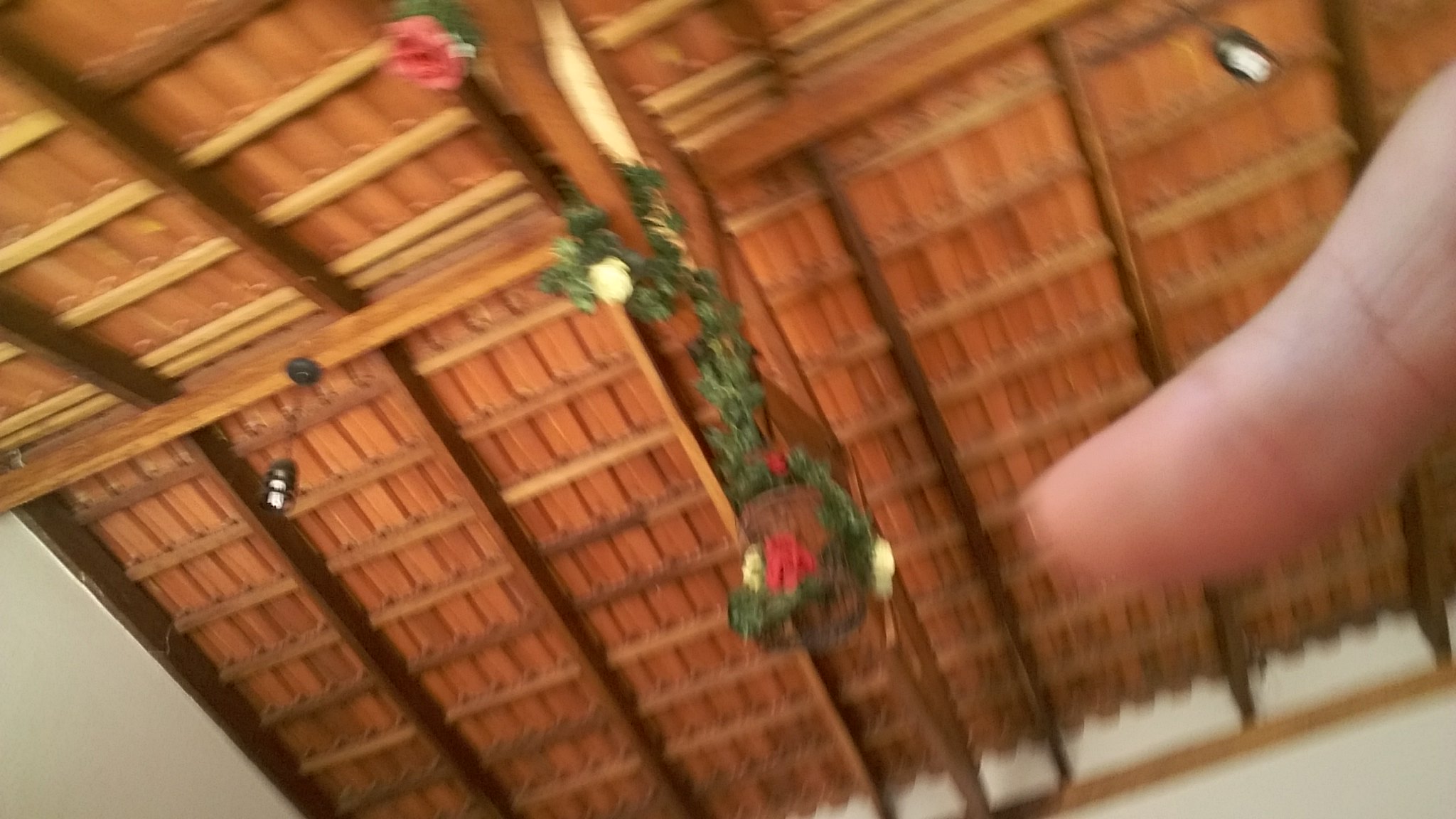The image captures a high wooden ceiling with a distinct frame structure and visible wooden slats. Hanging from the ceiling are two pendulum lights, positioned symmetrically on the left and right sides. Centrally located on the ceiling are festive Christmas decorations, adorned with green tinsel and a mix of red and white flowers, adding a touch of holiday spirit. On the right side of the image, there is a slightly blurry section, with a blurred finger, presumably of the photographer, partially obscuring that part of the view.